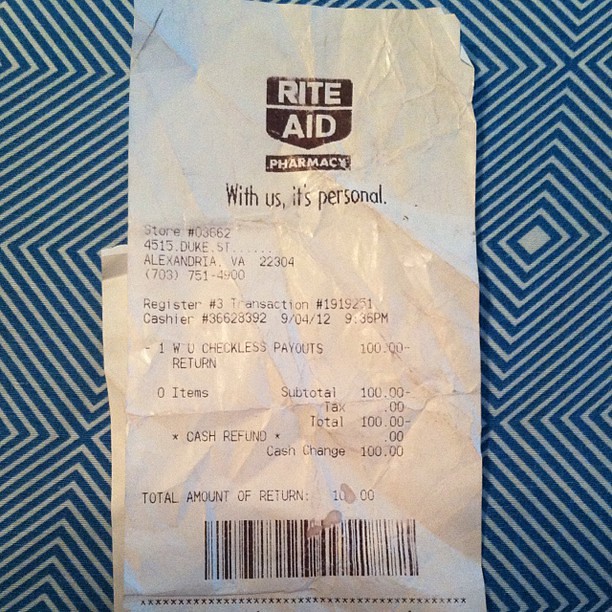The image features a vibrant pattern of blue and white stripes arranged diagonally. These stripes intersect in such a manner that they form a series of diamond shapes where the lines meet. The arrangement alternates directions, with some stripes running from the bottom left to the top right and others from the top left to the bottom right.

In the foreground of this patterned backdrop, there is a receipt from Rite Aid prominently displayed. The receipt's header lists "Rite Aid" at the top, followed by "Pharmacy" and their slogan, "With us, it's personal". Details include:

- Store Number: 03562-4515
- Location: Dukes Creek, Alexandria, Virginia, 22304-13703
- Phone: 751-4900
- Register Number: 3
- Transaction Number: 1919251
- Cashier Number: 36628392
- Slideshow: 412-9361
- Checklist Payouts: 100
- Return Item Count: 0

The financial summary at the bottom of the receipt shows:

- Subtotal: $100
- Tax: $0
- Total: $100
- Cash Rate: $10
- Cash Change: $100
- Total Amount of Return: $100

This image combines the geometric precision of the blue and white stripe pattern with the mundane detail of a typical store receipt, juxtaposing order and routine commerce.